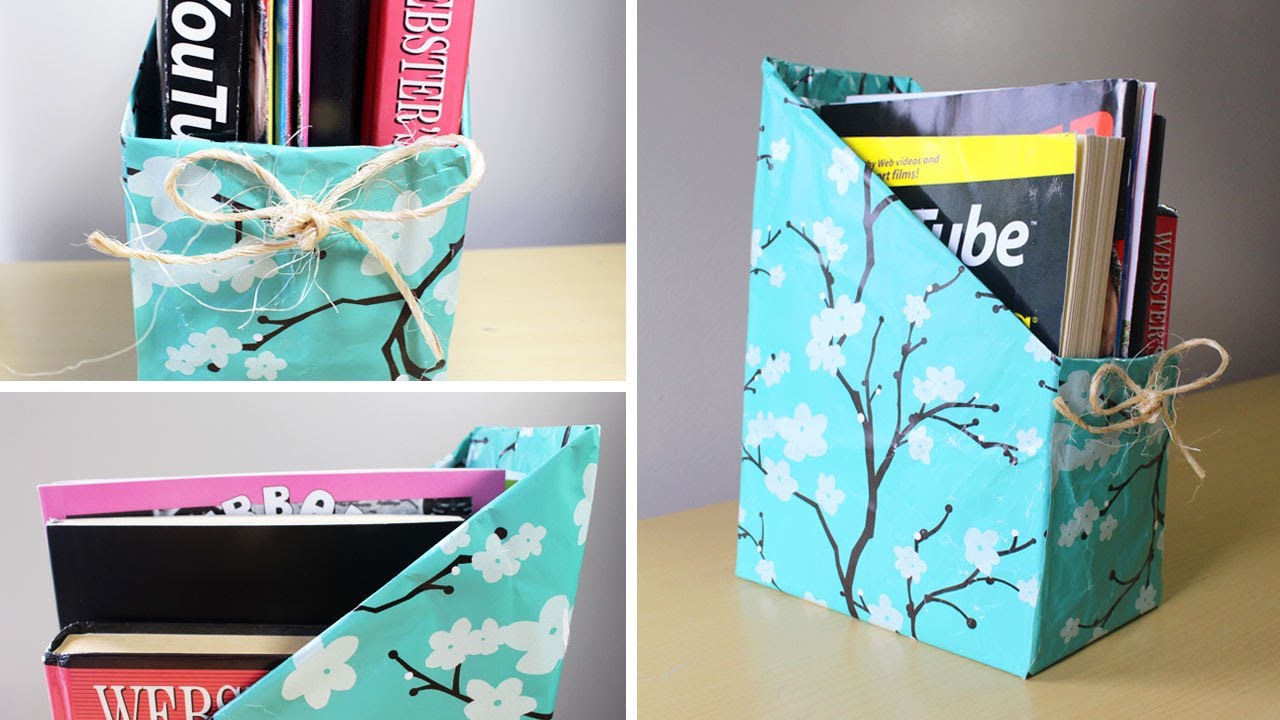This collage-style image showcases a handcrafted book holder from various angles, offering detailed insight into its design and functionality. On the left, the top image displays a blue floral-patterned container with white flowers and black stems, tied with a raffia ribbon. Inside the container, books are neatly stacked vertically. The bottom left image provides a close-up view of the topmost book's cover, revealing the text "W.E.R.S." The larger image on the right captures the entire container, highlighting its angled cut that facilitates easy reading of book titles, such as "T.U.B.E." This meticulously crafted book holder serves as an attractive and practical solution for organizing and displaying a small collection of books, perfect for a desk or interior decor.